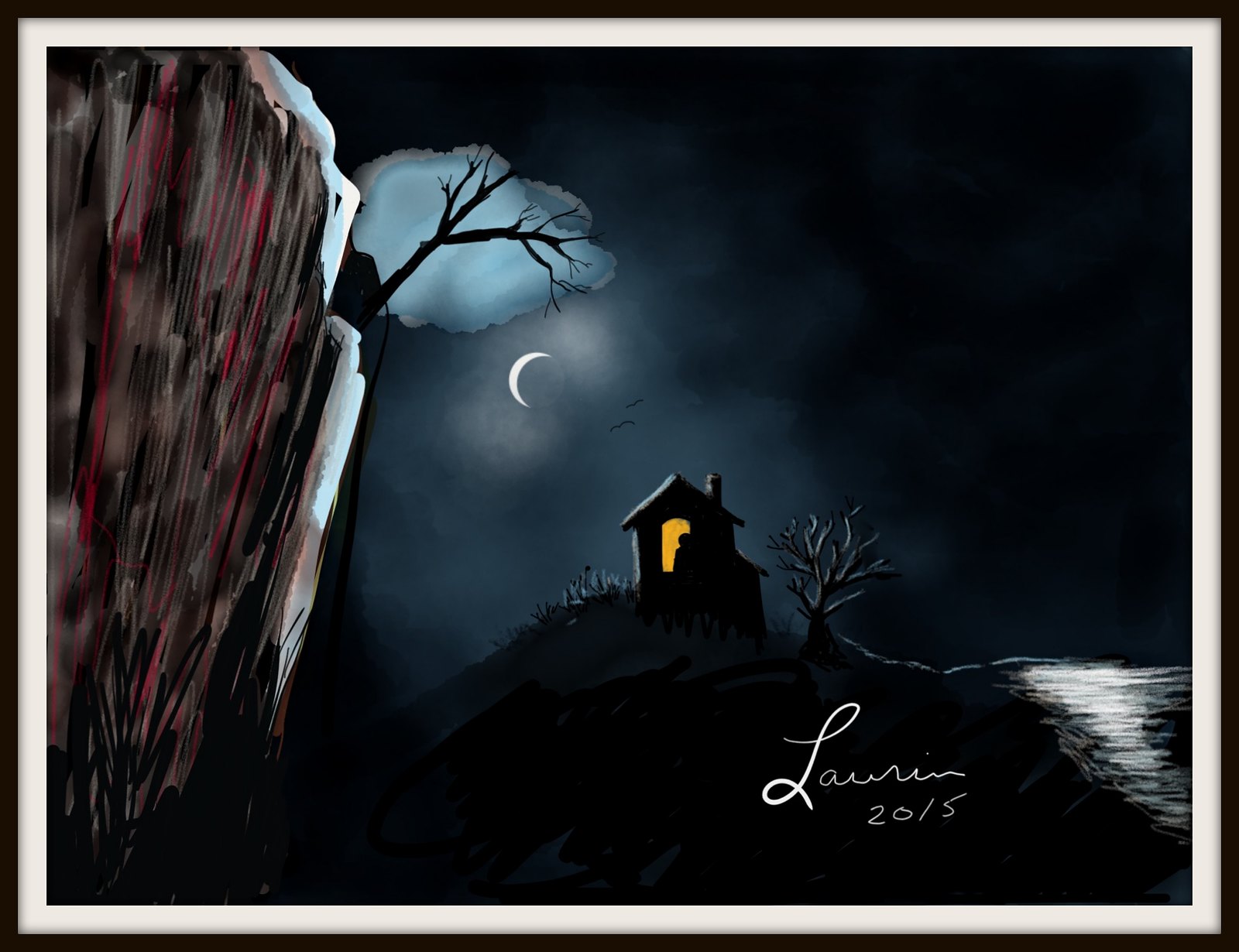A hand-painted postcard from 2015 by the artist Jamie features a dark, serene night scene by the ocean. The artwork, wider than it is tall, is framed by a crisp white border and includes the artist's handwritten signature in the bottom left corner. The composition is dominated by a cliffside on the far left, which occupies roughly a third of the width of the painting. A lone tree emerges from the top of the cliff, against a backdrop of a white cloud and a crescent moon. The moon's soft glow spreads a gentle light across the otherwise dark scene, creating the most illuminated area in the picture.

In the middle of the image stands a small, solitary house with a single yellow window, through which a person can be seen. Adjacent to the house is another tree, and to its right lies the tranquil ocean. The water reflects the moonlight in delicate white ripples, adding to the painting's sense of calm and introspection. Despite its simplicity, the composition powerfully evokes feelings of loneliness, peace, and tranquility, capturing a quiet, contemplative moment by the sea.